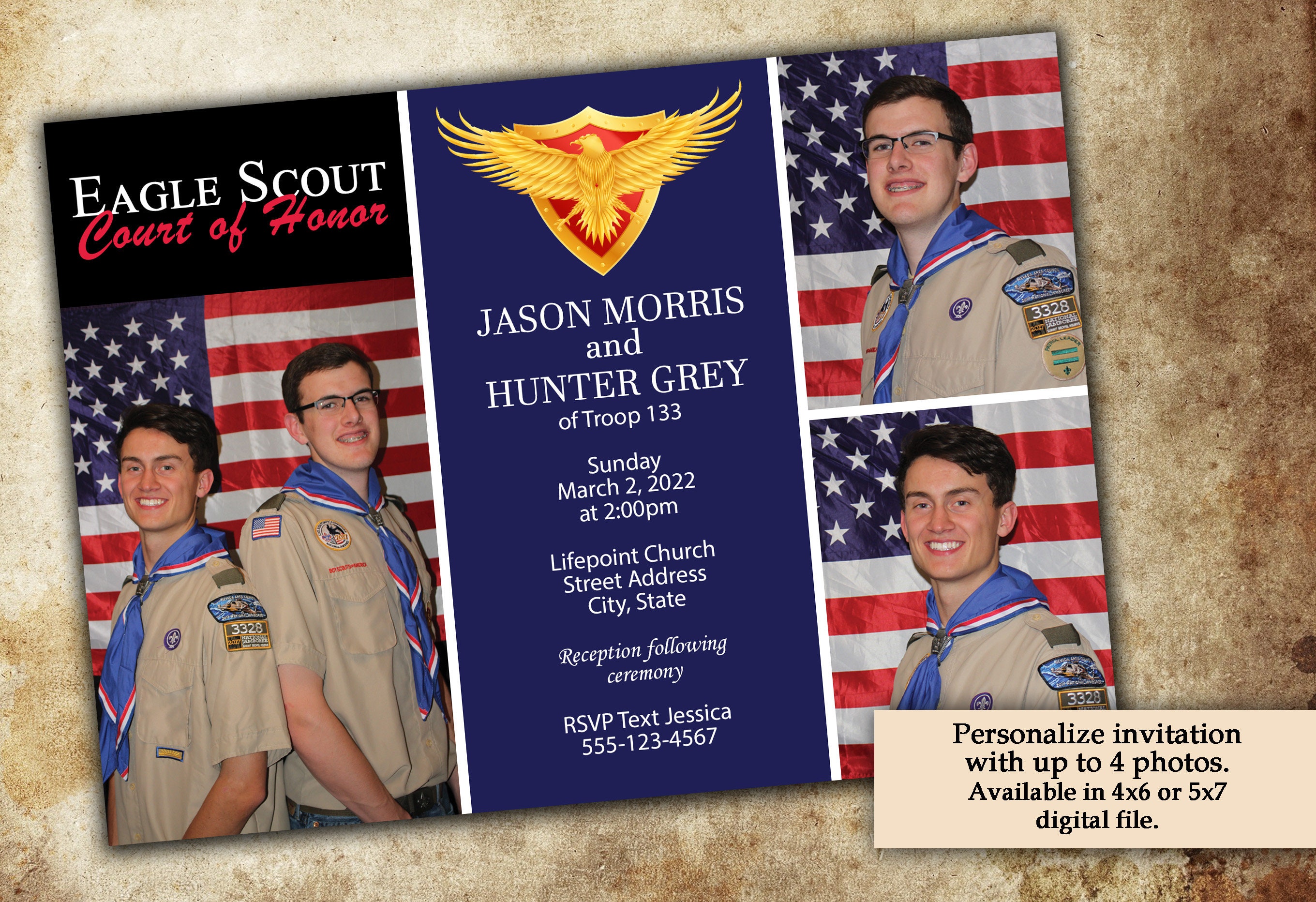The image is a detailed and personalized invitation for an Eagle Scout Court of Honor ceremony, designed as a foldable brochure divided into three sections. The left section features a photograph of two Eagle Scouts standing back-to-back, grinning, in front of a U.S. flag. They are dressed in khaki short-sleeved uniforms adorned with various badges and a blue, red, and white scarf knotted around their necks. The middle section is set against a blue background and includes an eagle shield emblem at the top. Text in white and red reads, "Eagle Scout Court of Honor." Below this, it announces, "Jason Morris and Hunter Gray of Troop 133," with event details, "Sunday, March 2, 2022, at 2 p.m. Life Point Church, [Street Address], [City, State]. Reception following ceremony. RSVP text Jessica at 555-123-4567." The right section displays additional individual photographs of the same two Eagle Scouts, each standing solo in front of the American flag, continuing the celebratory theme. At the bottom right, there is a note that this is a personalized invitation, available with up to four photos in 4 by 6 or 5 by 7 digital file formats.